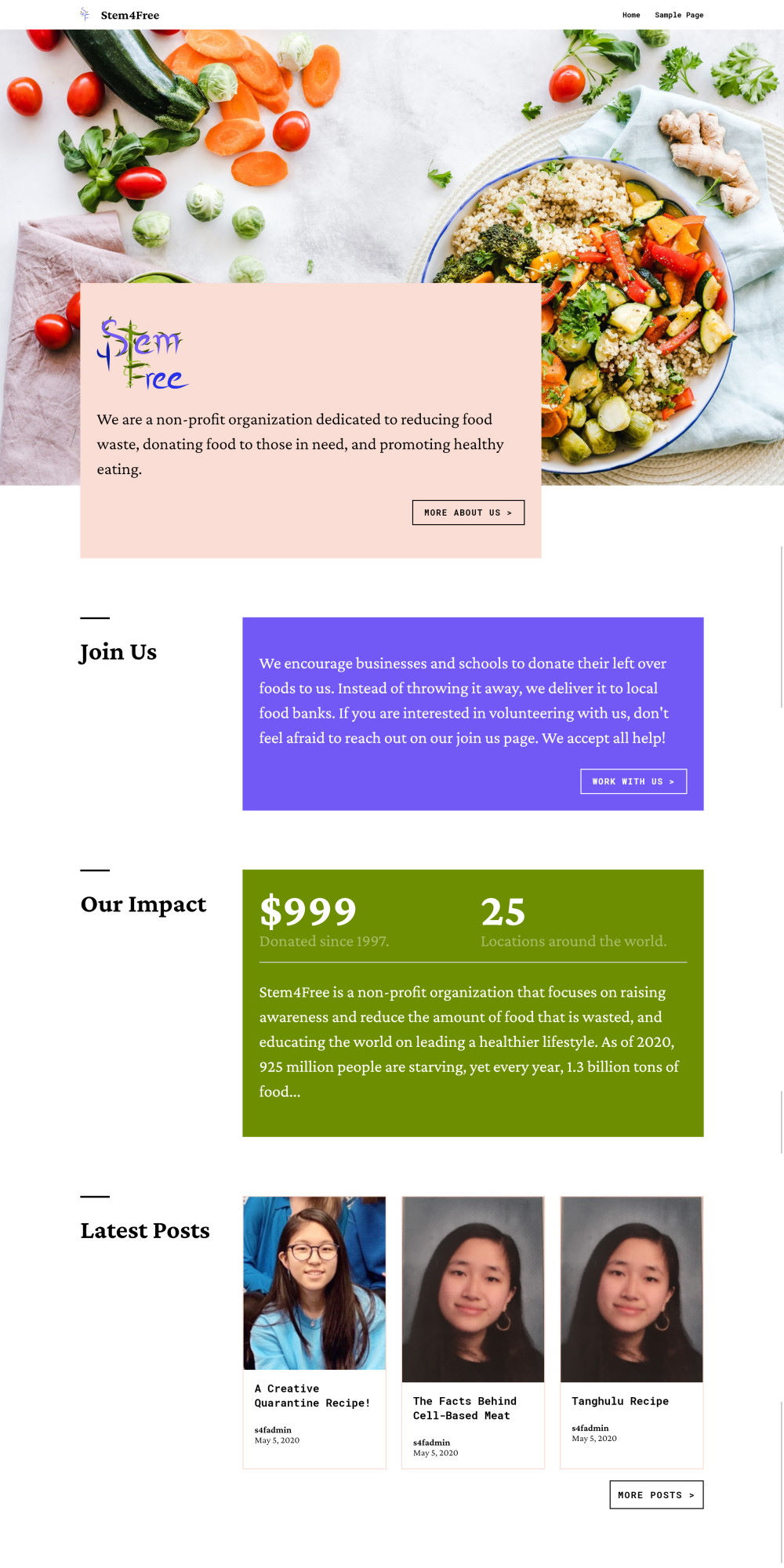The image showcases the homepage of the StemFree website. In the upper left-hand corner, the StemFree logo is prominently displayed. Below the logo is a top-down view of a dining table adorned with various items. Central to the table is a bowl filled with rice, chopped cucumbers, and possibly broccoli. The table is covered with a white cloth, and scattered across it are cherry tomatoes and a partially visible zucchini entering from the top left corner. Towards the bottom left-center of the table, a light pink box labeled "StemFree" states, "We are a non-profit organization dedicated to reducing food waste, donating food to those in need, and promoting healthy eating." The website is divided into three main sections: "Join Us," "Our Impact," and "Latest Posts."